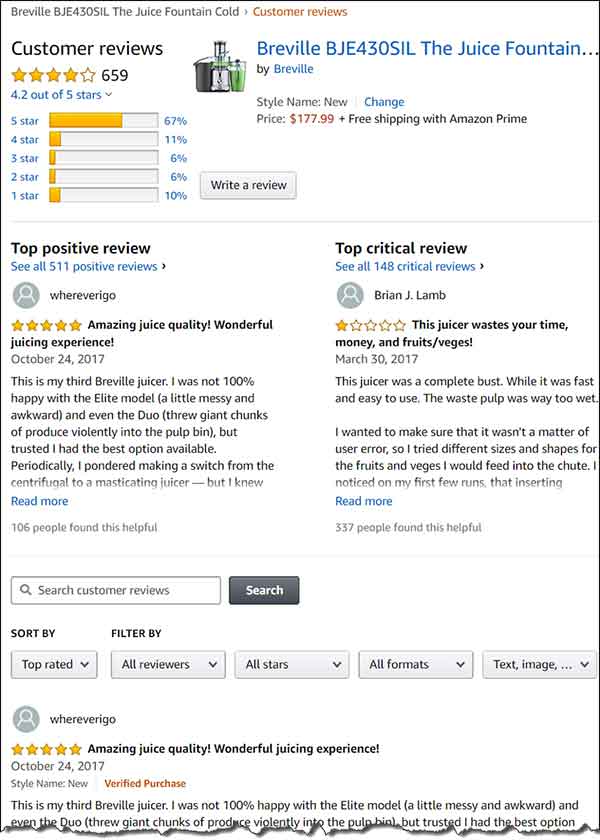Detailed Caption for the Image:

The image depicts a comprehensive snapshot of customer reviews for the Breville BJE430SIL Juice Fountain Cold on an e-commerce site. At the top, a heading reads "Breville BJE43OSIL, Juice Fountain Cold Customer Reviews," followed by the overall rating of 4.2 out of 5 stars. This rating is visually represented by four fully colored-in stars. The total number of reviews stands at 659, with a detailed breakdown: 67% are 5-star reviews, 11% are 4-star reviews, 6% each are 3-star and 2-star reviews, and 10% are 1-star reviews.

On the right-hand side, there's an image of the Breville BJE430SIL Juice Fountain. Alongside, it's noted that the juicer is a "New" style, priced at $177.99 with free shipping available via Amazon Prime.

Below this section, there’s an area highlighting both the top positive and top critical reviews. The top positive review is by a user named "wherever I go," who rated the juicer 5 stars, praising the amazing juice quality and wonderful juicing experience in a review dated October 24, 2017. They mention this is their third Breville juicer, expressing some dissatisfaction with earlier models but ultimately trusting Breville's quality. This review has been marked helpful by 106 people, and there's a "read more" link for further details.

Conversely, the top critical review is by "Brian J. Lam," who gave the juicer just 1 star in a review dated March 30, 2017. He criticizes the juicer for wasting time, money, and produce, complaining about the overly wet waste pulp despite trying different methods. This review has been marked helpful by 337 people and also includes a "read more" link for additional content.

Below the reviews section, there's a search box enabling users to search customer reviews, along with sortable filters labeled "Sort By" and "Filter By," which include options like top rated, all reviews, all stars, all formats, text, and image.

The bottom of the page has an aesthetic resembling a torn or ripped edge, giving the screenshot an unfinished look.